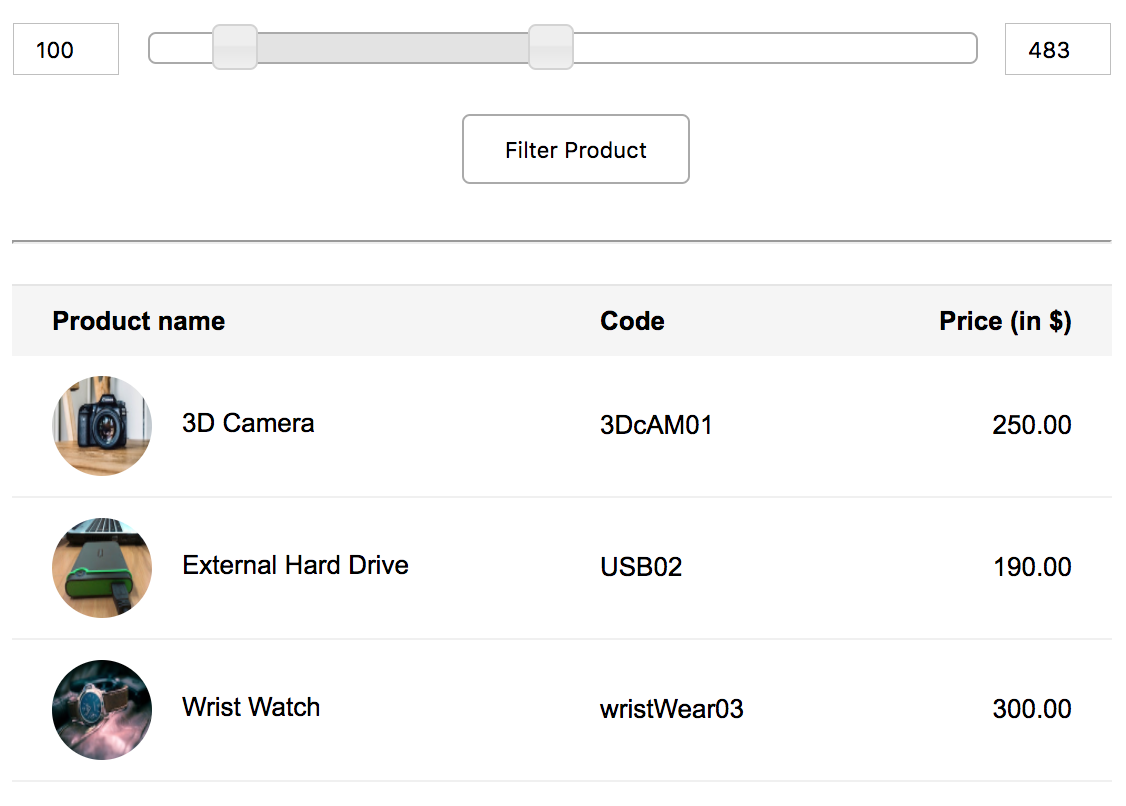The screenshot displays a navigation bar at the top. On the left side of this bar, there is a boxed number "100," and on the right side, a boxed number "483." The bar itself starts with a white section, transitions into a purple section bounded by a box, and then reverts to white leading up to the "483."

Below this navigation bar, there is a clickable option labeled "Filter Product." In bold text against a purple stripe, there are black inscriptions that read "Product Name," "Code," and "Price in Dollars."

Three products are listed below this heading:
1. **3D Camera** – Accompanied by an image of a camera, priced at $250.
2. **External Hard Drive** – Showcasing a green hard drive, priced at $190.
3. **Wrist Watch** – Featuring a wristwatch with a brown leather band, priced at $300.